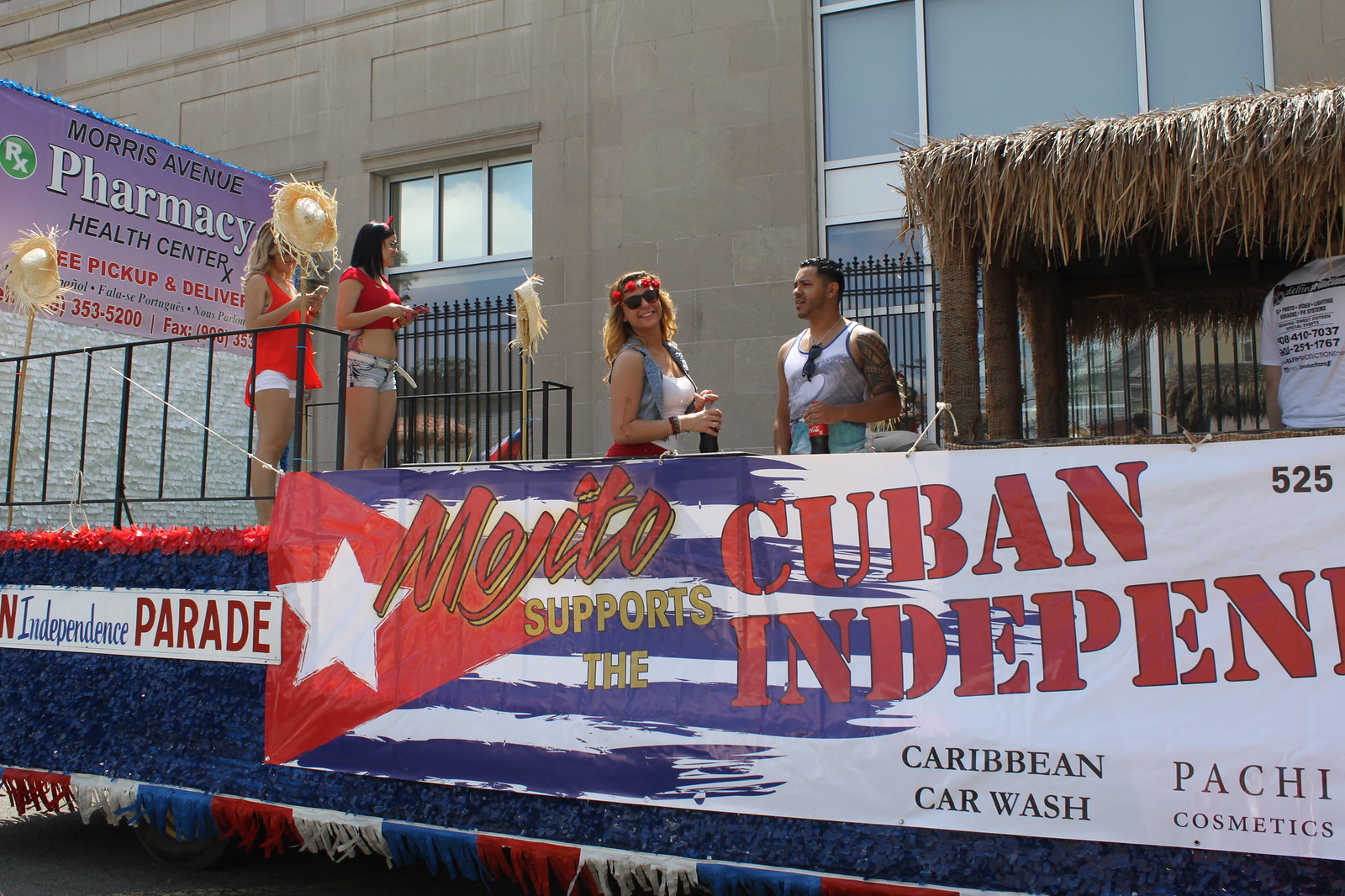In a vibrant outdoor parade celebrating Cuban independence, a colorful float cruises past a tan and white-brick building. On this float, a tiki hut style gazebo adds a festive touch amidst a sea of red, blue, and white decorations. At the forefront, a large sign reads "Mojito supports the Cuban independence," with an artistic rendition of a Cuban flag beneath it. The float carries a spirited group: three women and one man. One woman, wearing a red midriff shirt and shorts, stands with another woman in a red flowy tank top and white shorts, both engrossed in their phones. Further to the right, a woman in a red floral headband, sunglasses, and a sleeveless jean jacket holds a Coca-Cola beside a man in a tank top with sunglasses dangling from the collar. Behind the float, a banner advertises "Morris Avenue Pharmacy Health Center," set against a purple background offering free pickup and delivery services. The energy of the Cuban independence movement fills the daytime air, with each participant adding to the celebratory atmosphere.